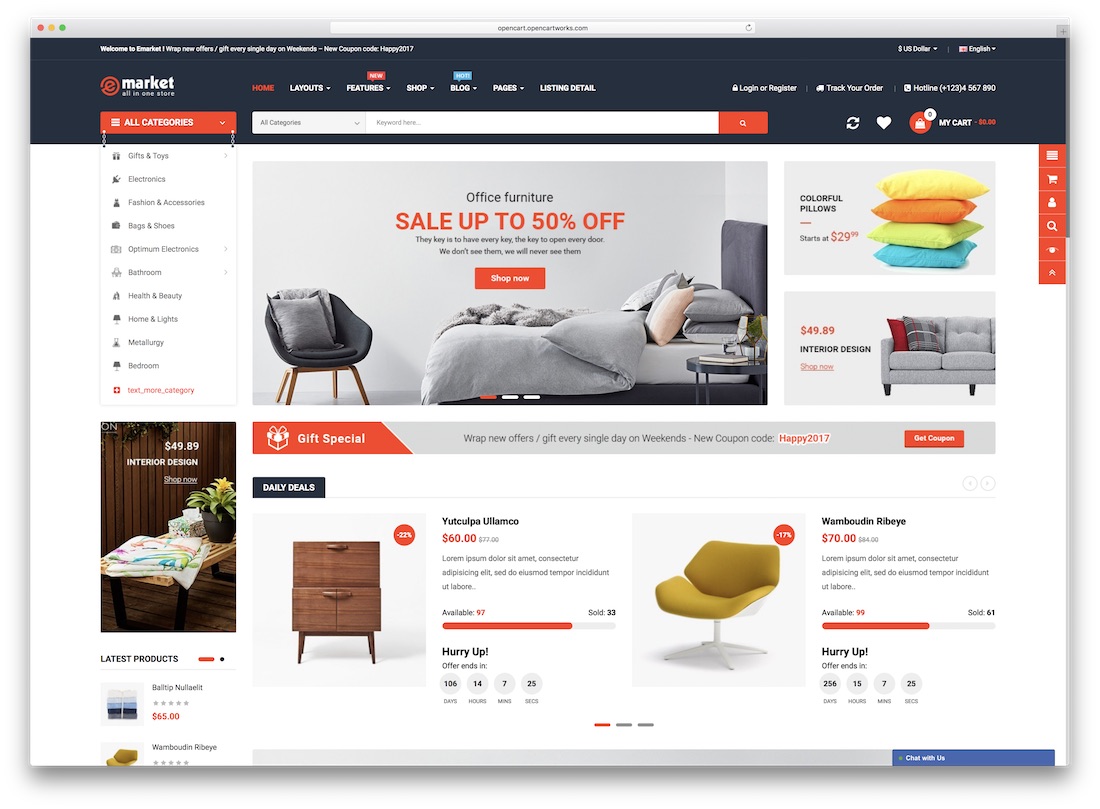A detailed screenshot captures a mock website viewed on a laptop or desktop's computer browser, highlighting the layout and design elements distinctly suited for larger screens compared to mobile browsers. The focal point of the website is its black header, which occupies roughly 12% of the screen space. Within this header, a stylized logo featuring a red "E" encapsulated in a circle, followed by the word "Market" in white, and additional smaller white text presumed to be a tagline, stands prominent. This could either be a significant branding element or merely a placeholder.

Accompanying the logo are various navigation options, though their labels are not entirely legible. Adjacent to these options is a comprehensive search bar allowing users to search across all categories. The search interface includes a text input area and a distinct search button marked by a white magnifying glass on a red background. In the corner of the header, there appears to be contact information resembling a phone number, alongside what could be currency and language selection options.

The website's body is divided into a two-column layout. The left-side column functions as a menu, listing the latest products and special items along with navigational links. The right-side column serves as the main content area. This area starts with special announcements prominently displayed at the top, transitioning into a section for daily deals. Featured here are two meticulously chosen mid-century furniture pieces, exemplifying the type of products the website intends to showcase.

Overall, this mock website design integrates both usability and aesthetic components, creating an organized, navigable interface for an enhanced user experience.